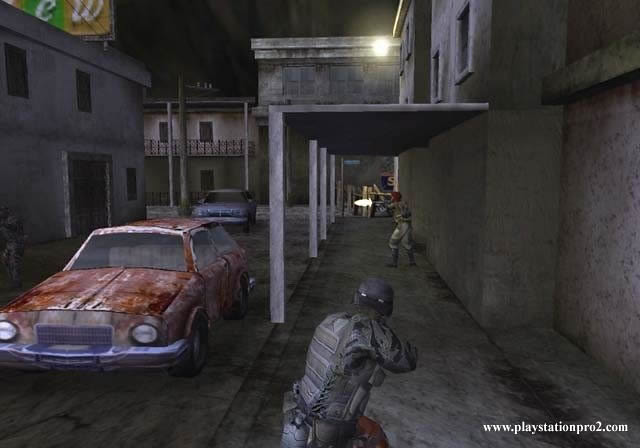This screenshot capture is from what appears to be either a first-person or third-person military shooter game. The scene is set in a dilapidated town, characterized by its rundown buildings and barren streets. Two soldiers are featured prominently in the image, fully clad in standard military attire and gear, positioned within the town's desolate environment. The overall color palette of the scene leans heavily towards muted greys and browns, a result of the low-quality textures on both the buildings and the ground, giving the atmosphere a somber and gritty feel. In the bottom right corner, the text "playstation2pro.com" is visible, likely indicating the source or platform related to the game.